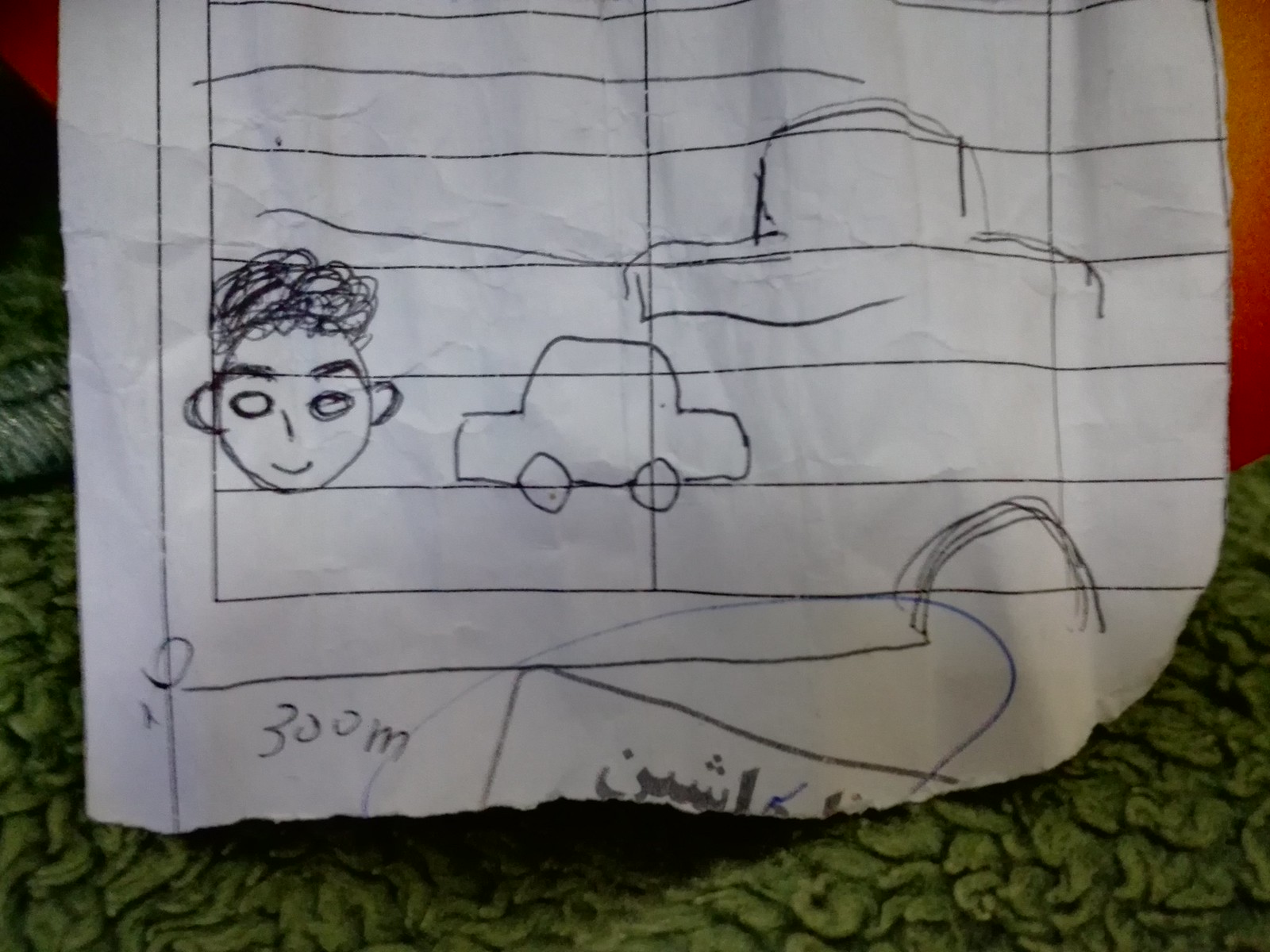The image showcases a piece of torn grid paper featuring various doodles. The paper is visibly ripped along the sides and bottom edge, giving it a rugged appearance. The grid pattern indicates that it was originally blank grid paper. On the bottom left corner, there's a detailed doodle of a face characterized by tall, circular hair on top and bald sides. The eyebrows are thick and shaded with pencil, and the ears and eyes are outlined multiple times with a black ink pen, creating a repetitive circular pattern. The face has a minimalistic line for the nose and a simple "U" shape for the mouth.

Moving to the center bottom of the page, there's a doodle of a car. Its shape resembles a hat on wheels, with a rounded top and rectangular sides. To the right of this smaller car, there’s a larger, more detailed attempt at drawing a similar car, maintaining the same overall shape and features. At the very bottom of the page, the text "300M" is written, and further to the right, there's a section of text that appears to be Turkish, written at an angle.

The piece of paper is positioned against an orange item, pieces of which are visible at the top right and left corners of the image. The background features a green rug or carpet that appears matted down, adding texture and context to the scene.